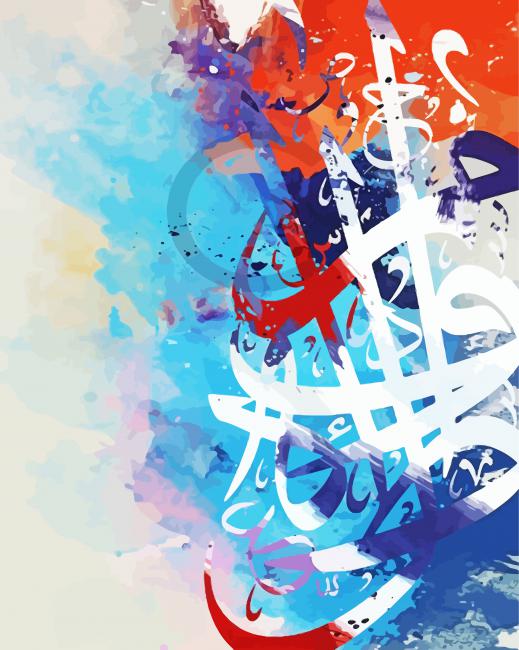The image depicts an abstract painting with a vibrant, chaotic interplay of colors and shapes. The left side features a subdued palette with hues of gray, light blue, light purple, and light yellow blending together in a watercolor-like effect. Meanwhile, the right side bursts into a dynamic display of predominantly white ribbons swerving erratically across the canvas, intersected several times by vigorous horizontal slashes. This area is marked by bold, broad sweeps of red, blue, and colorful accents including splashes of orange and dark purple. At the top, the colors transition into intense reds and oranges, while the bottom shows hints of blue. The painting evokes a sense of wild creativity, as if the colors themselves were alive, merging and colliding in unpredictable patterns.